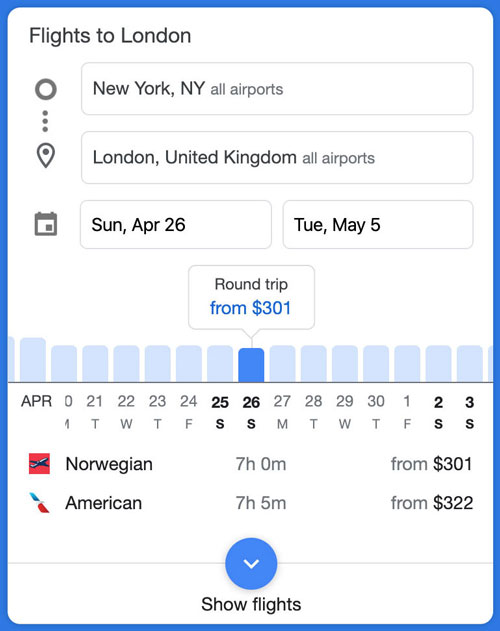This image displays a flight booking website, framed with a blue border, showcasing flight options to London. At the top, large, bold text reads "Flights to London."

Below that, two search bars allow users to input their departure and arrival locations. The departure field is filled with "New York, New York, all airports," while the arrival field is set to "London, United Kingdom, all airports."

Following the search bars, there are two date selection boxes for entering the departure and return dates, each featuring a small calendar icon for user convenience. The selected dates are from Sunday, April 26th to Tuesday, May 5th.

Beneath these fields, a highlighted box advertises "Round trip from $301," emphasizing an attractive fare.

A timeline with blue date boxes spans the section below, marking available travel dates from April 21st to May 3rd. The interface offers carrier options, including a Norwegian airline marked with a red box and an airplane icon, and an American airline option adjacent to it.